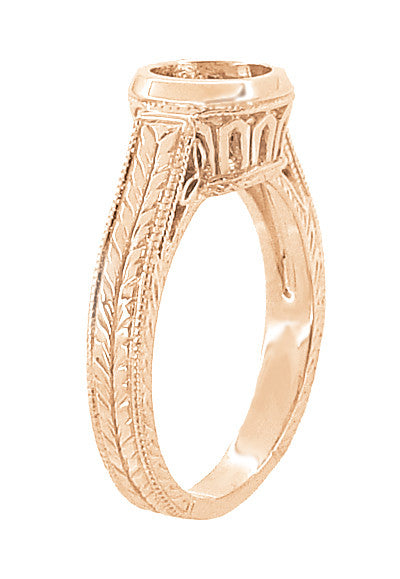This image features a detailed close-up of an intricately carved vintage art deco ring. The ring, displayed vertically against a solid white background, is composed of gold, though it has a bronze-like appearance in parts. The band’s interior is smooth, contrasting with the elaborate design on the outside, which showcases a wheat pattern and arches engraved into the metal. The most distinctive feature is the empty round setting at the ring’s top, where a jewel, such as a diamond, is typically inlaid. In this particular image, the hole meant for the gem is vacant, revealing more of the ornate craftsmanship that adorns the ring.